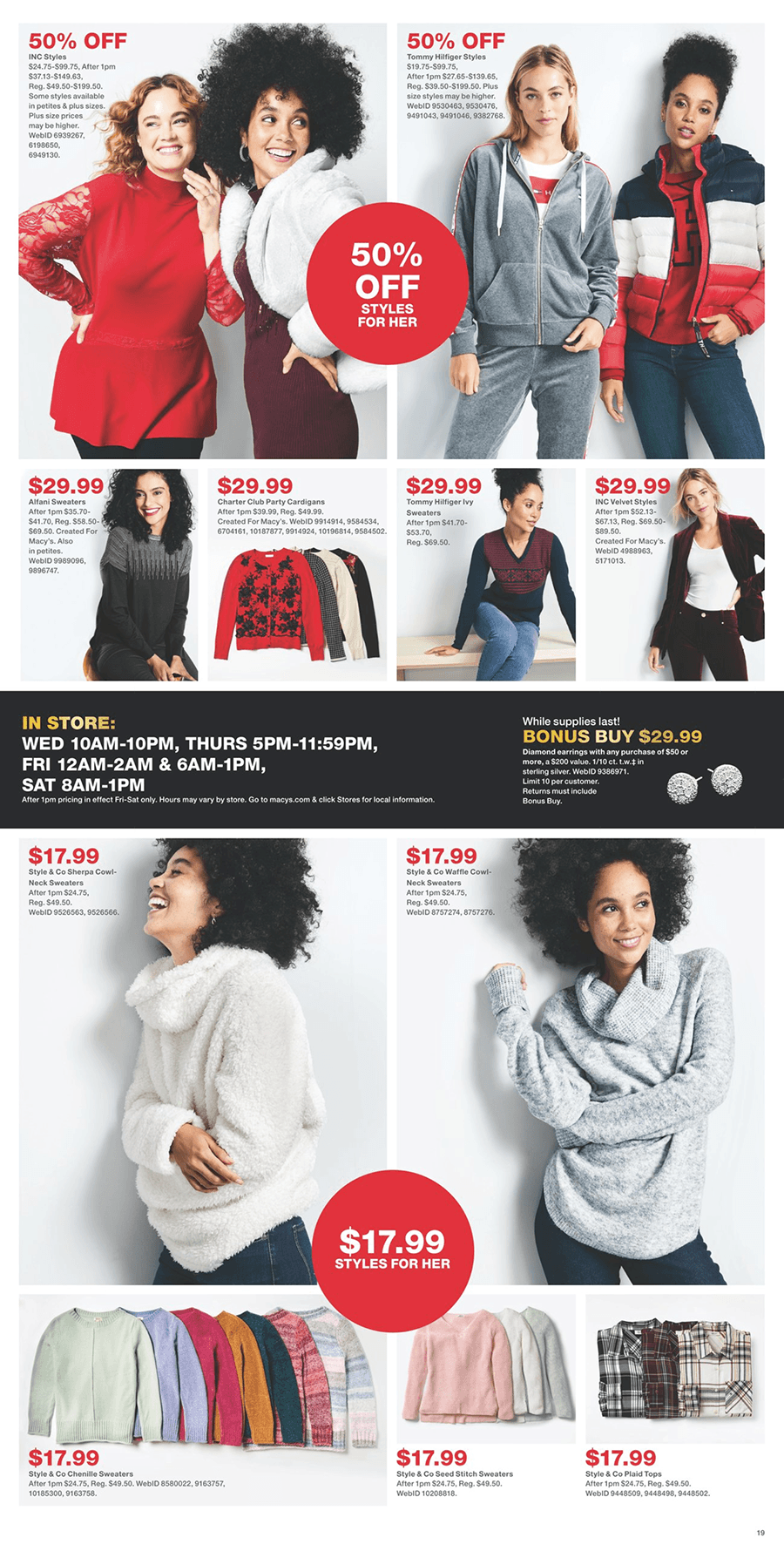Introducing our latest Macy's Fall Fashion Sale! Featured on this vibrant sales page are stylish selections you'll love, all at 50% off!

At the top left, we have a stunning duo. The first model, a light-skinned Black woman with a voluminous curly afro, exudes elegance in a white faux fur coat layered over a burgundy dress. Beside her, a white woman with fiery red shoulder-length hair and in her 30s, adds a touch of sophistication with her red lace-sleeved top paired with sleek black pants.

In the top right section, two more chic looks await. A white woman with dark blonde hair rocks a casual yet trendy gray tracksuit featuring white and red stripes on the sleeves. Alongside her, a light-skinned Black woman with her hair styled in a high pony puff, brings sporty flair with a red, white, and blue Tommy Hilfiger puffer jacket, a red T-shirt, and fitted jeans.

Dominating the center of the page, a bold headline announces, "50% Off Styles for Her," highlighting the incredible savings.

Moving to the bottom, discover even more fabulous finds. One ad showcases a light-skinned Black woman modeling a white cowl-neck sweater, priced attractively at $17.99. Beside her, another black woman, in a cozy gray cowl-neck sweater, also available for just $17.99.

Don't miss out on these phenomenal deals on INC and Tommy Hilfiger styles, exclusively at Macy's!